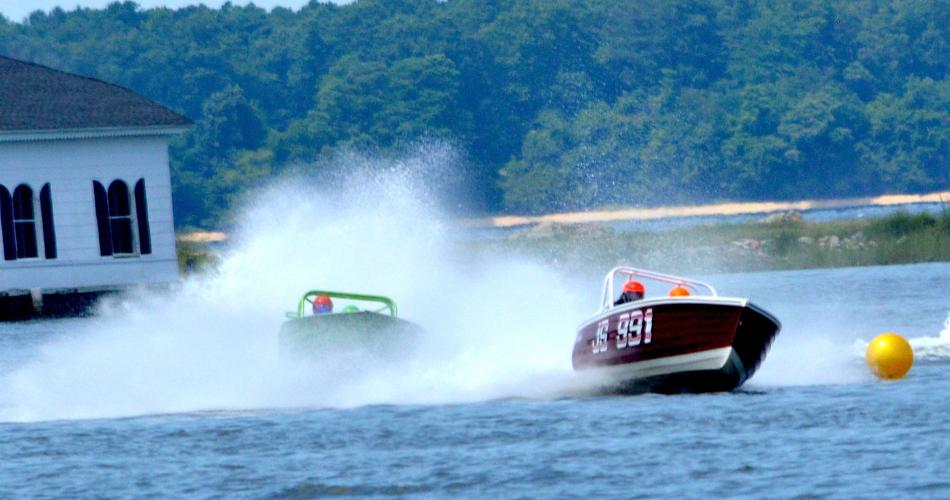The image features an exhilarating race between two speedboats jetting across a lake, creating significant splash clouds as they speed along. The boat in the lead is a sleek black vessel with a white bottom, prominently marked with the number "JS 991" in white text. This boat is rounding a gold flotation marker on the right side of the image. Trailing behind is a green speedboat, also with a white bottom and a green roll bar, which is partially obscured by the water spray from the boat ahead. Both racers are wearing red helmets. In the upper left corner of the image, a white boathouse with a black roof and windows can be seen. Dense green forest occupies the upper portion of the background, adding natural serenity to the high-speed action below. The contrast of the disruptive water sprays and the calmness of the surrounding environment captures the dynamic and thrilling nature of the race.